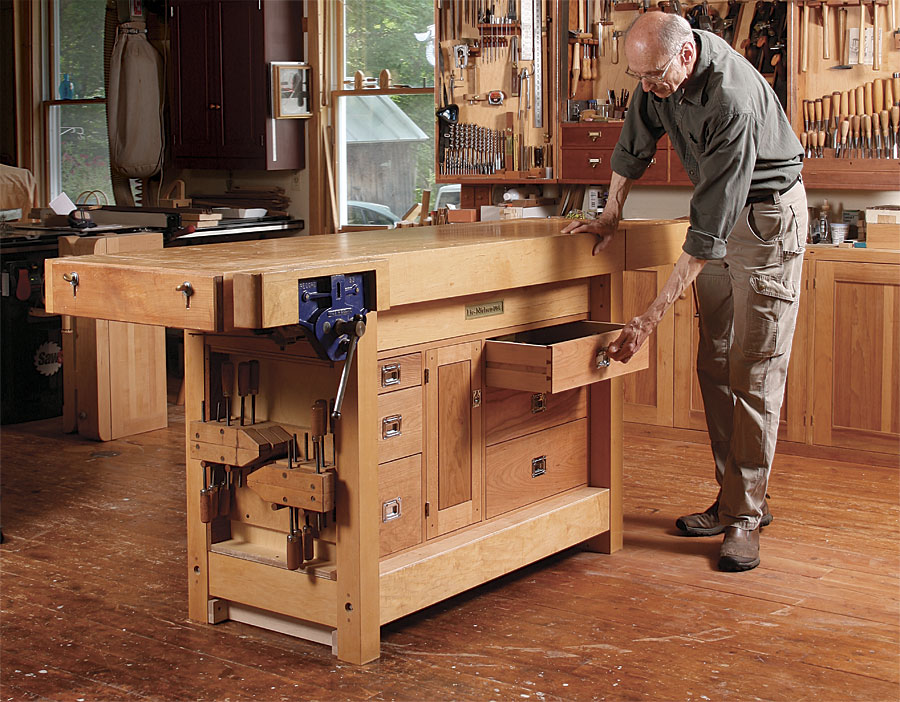The photo captures an older gentleman, approximately 60-65 years old, in a pristine woodworker's studio. He has a balding head with gray hair at the sides, wears wire-rim glasses, a rolled-up green long-sleeved shirt, beige cargo pants, and brown shoes. He is leaning over a modern, light brown workbench with his right hand placed on it while his left hand opens a dovetail drawer, showcasing the exceptional craftsmanship. The workbench, equipped with a large stainless steel handled blue vise on the side, appears new and includes several drawers and tool storage features. The studio has a well-worn wooden plank floor, indicating extensive use, and is well-lit with several windows providing natural light and a view of another outbuilding. The background is lined with wooden cabinets filled with various woodworking tools, including hammers, chisels, and drill bits, all meticulously organized, contributing to the ambiance of this fine craftsmen's workshop.